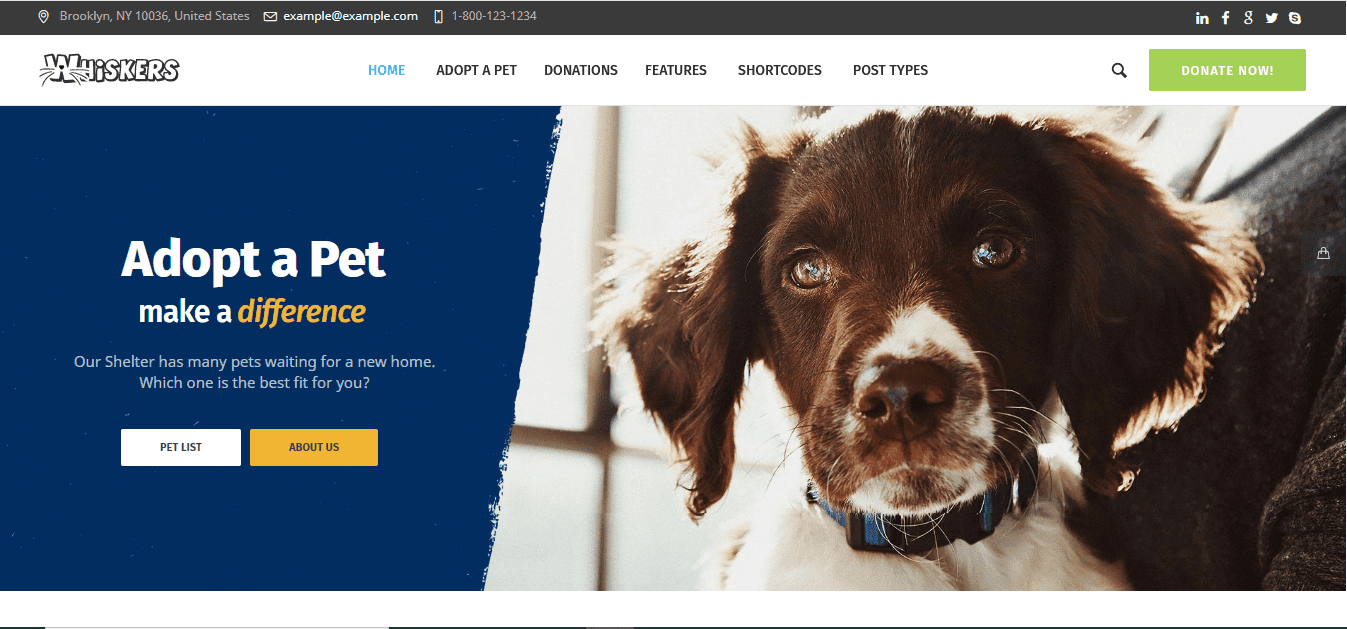**Website Screenshot Description:**

At the top of the screenshot is a charcoal black navigation bar displaying essential contact information in white font. The information includes the location "Brooklyn, New York 10036, United States," followed by an email address "example@example.com" and a phone number "1-800-123-1234." To the right, there are social media icons for Google, Twitter, and Facebook.

Below this navigation bar, a white bar features prominently. On the left side of this bar, the site’s name, "Whiskers," is displayed in playful bubble letters, with whisker details creatively integrated into the "W." Next to the site name, there are several navigation options in a horizontal menu: "Home" (highlighted in blue to indicate it’s the selected page), "Adopt a Pet," "Donations," "Features," "Short Codes," and "Post Types," all written in black font. A black magnifying glass icon for search functionality is also present.

On the right end of the white bar, there's a green button with white text that reads "Donate Now!" 

Below this white bar, the main image shows an adorable Springer Spaniel puppy. The puppy has a predominantly black head with a bit of white on its muzzle, and a white chest, radiating cuteness and charm.